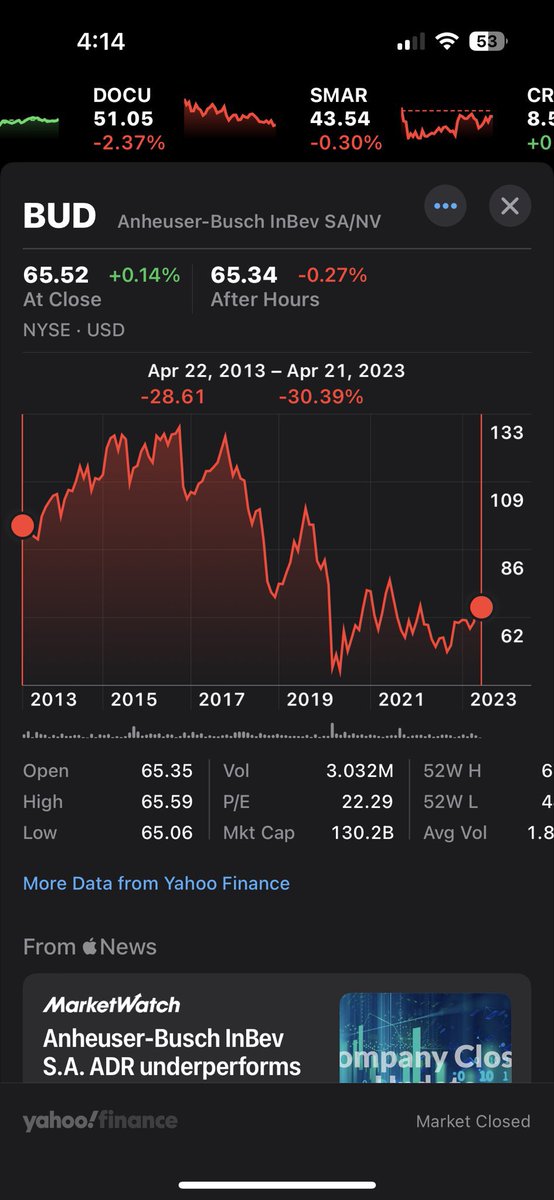The image displays a financial stock tracking application on a mobile device with a black background. At the top of the screen, the status bar shows the time (4:14), signal strength, Wi-Fi connection, and battery charge levels.

Beneath the status bar, there is a list of stocks being tracked. The entries include:
- DOCUSMAR: DOCU listed at $51.05 (down 2.37%), and SMAR listed at $43.54 (down 0.3%).

Following this, more detailed information is provided for Anheuser-Busch InBev, indicated as “Bud”:
- At close: $65.52 (up 0.14%).
- After hours: $65.34 (down 0.27%).
This stock is traded on the New York Stock Exchange (NYSE) and prices are in U.S. dollars.

Below this, a graph displays the historical performance of Anheuser-Busch InBev stock from April 22, 2013, to April 21, 2023. Annotated changes show a decline of 28.61% and 30.39%. The graph itself includes time on the horizontal axis and what is presumed to be the stock price on the vertical axis.

Further details listed under the graph include metrics such as open, high, low, volume, P/E ratio, market cap, 52-week high and low, and average volume.

At the bottom of the screen, there is a blue link for additional data from Yahoo Finance. Supplementary news from Apple News highlights a MarketWatch article about Anheuser-Busch InBev's performance, noting the stock "underperforms."

This comprehensive caption captures the content and structure of the financial tracking application with extensive detail.